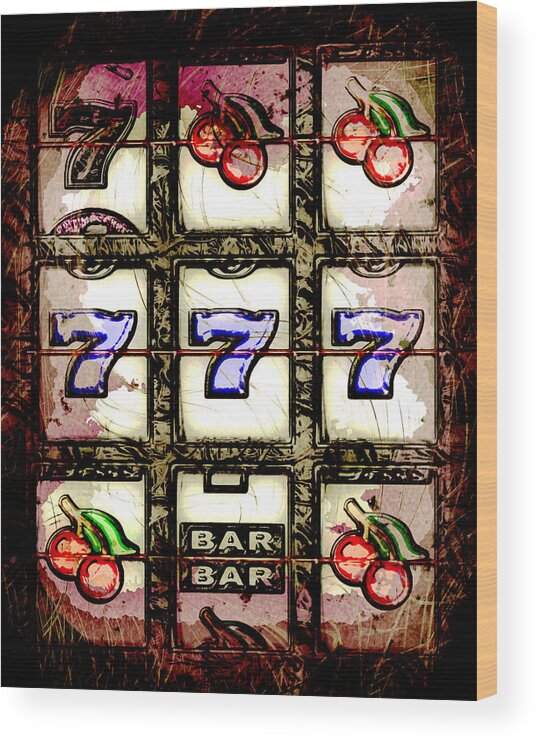This image is a detailed painting of a classic, non-digital slot machine expertly rendered on a light wooden plank. The wooden surface, partially visible at the edges, serves as the backdrop for the painted slot machine. The slot machine illustration spans three rows, each consisting of three sections, mirroring old-school mechanical slot machines typically found in casinos.

The top row features a black number seven paired with two cherries, vividly colored to enhance their nostalgic charm. The middle row showcases three bluish-white sevens in a line, highlighted by a distinctive cross line that connects them. Finally, the bottom row displays a cherry in the first box, a "BAR BAR" symbol in the second, and another cherry in the third box, again with a crossing line that ties the elements together.

The entire painting is structured within a dark brown border that imparts a metallic appearance, though the medium is unmistakably painted wood. The cherries are notably detailed, complete with red fruit and green stems, adding a touch of realism to the stylized artwork. This dreamily styled painting, likely designed to be hung on a wall like a picture, exudes a vintage aesthetic, meticulously crafted to evoke the timeless allure of classic slot machines.